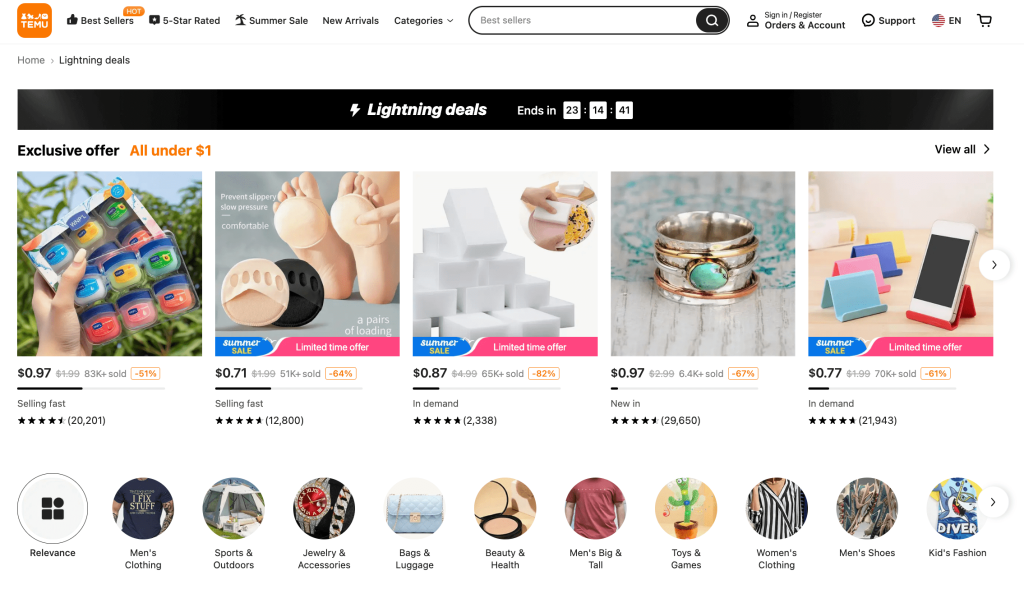**Caption:**

A detailed screenshot of the T-Moon online marketplace interface reveals a user navigating the "Lightning Deals" page. The top navigation bar prominently displays T-Moon's logo on the far left, followed by a series of clickable options including Bestsellers, Five-Star Ratings, Summer Sale, New Arrivals, and a drop-down menu for Categories. Adjacent to these options is a search bar, allowing users to input specific search inquiries. Further to the right, users have access to sign-in/register options, order and account information, and a support button. Additionally, there's a language selection feature, currently set to English, followed by a heart icon.

The "Lightning Deals" banner, positioned centrally, highlights that the deals end in 23 hours, 14 minutes, and 41 seconds. Beneath the banner, exclusive offers for items priced under a dollar are presented. Each item displays an image, price, the amount sold, the discounted percentage, and the number of reviews. Visible items include a container of Vaseline, foot slippers or a pressure-relief device for the balls of one's feet, multi-use sponges, a distinctive ring, and phone holders.

Below these featured deals, there are clickable sections leading to different parts of the website, including Clothing, Toys, Beauty & Health, and more, indicated by additional item images.